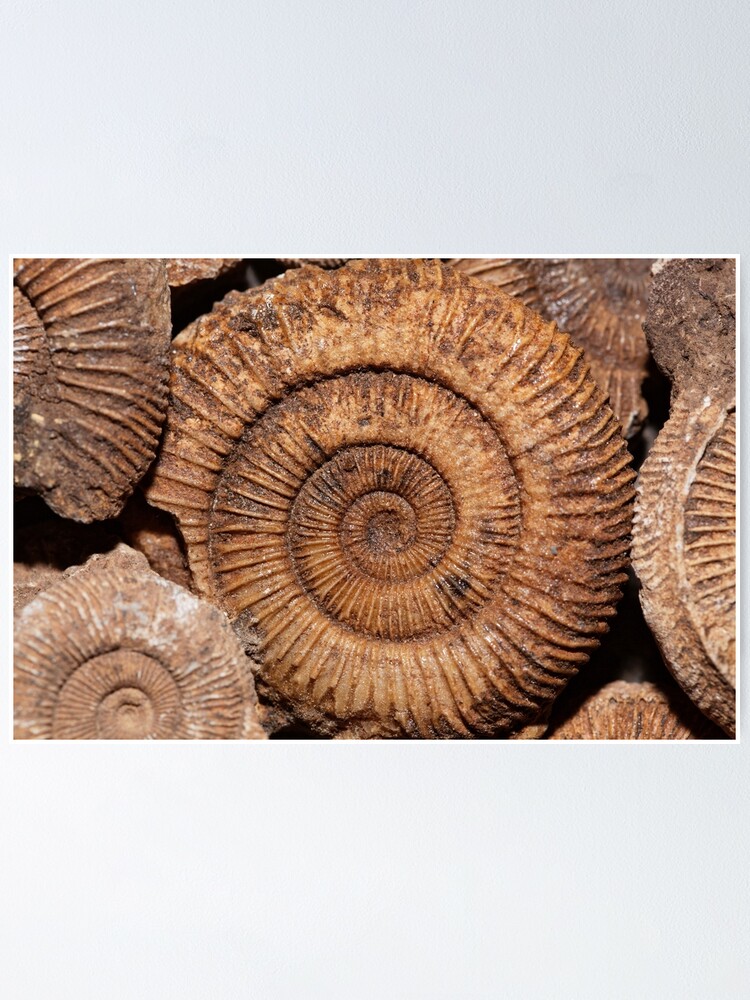This close-up photograph showcases a collection of fossilized, spiral-shaped seashells in various shades of brown, ranging from rust to tan with hints of gray, orange, and black. Dominate in the center is a nearly intact, round fossil that spirals inward with detailed ridges along its surface. This central fossil has a minor break on its bottom left side. Surrounding it, the background features multiple, similar fossils — slightly lighter in tone, including a smaller one on the bottom left, a broken, darker one on the top left, and half of another visible towards the right. The assortment of these rigid, ancient shells, some broken and fragmented, gives the image a rich texture, reminiscent of discoveries on a beach.